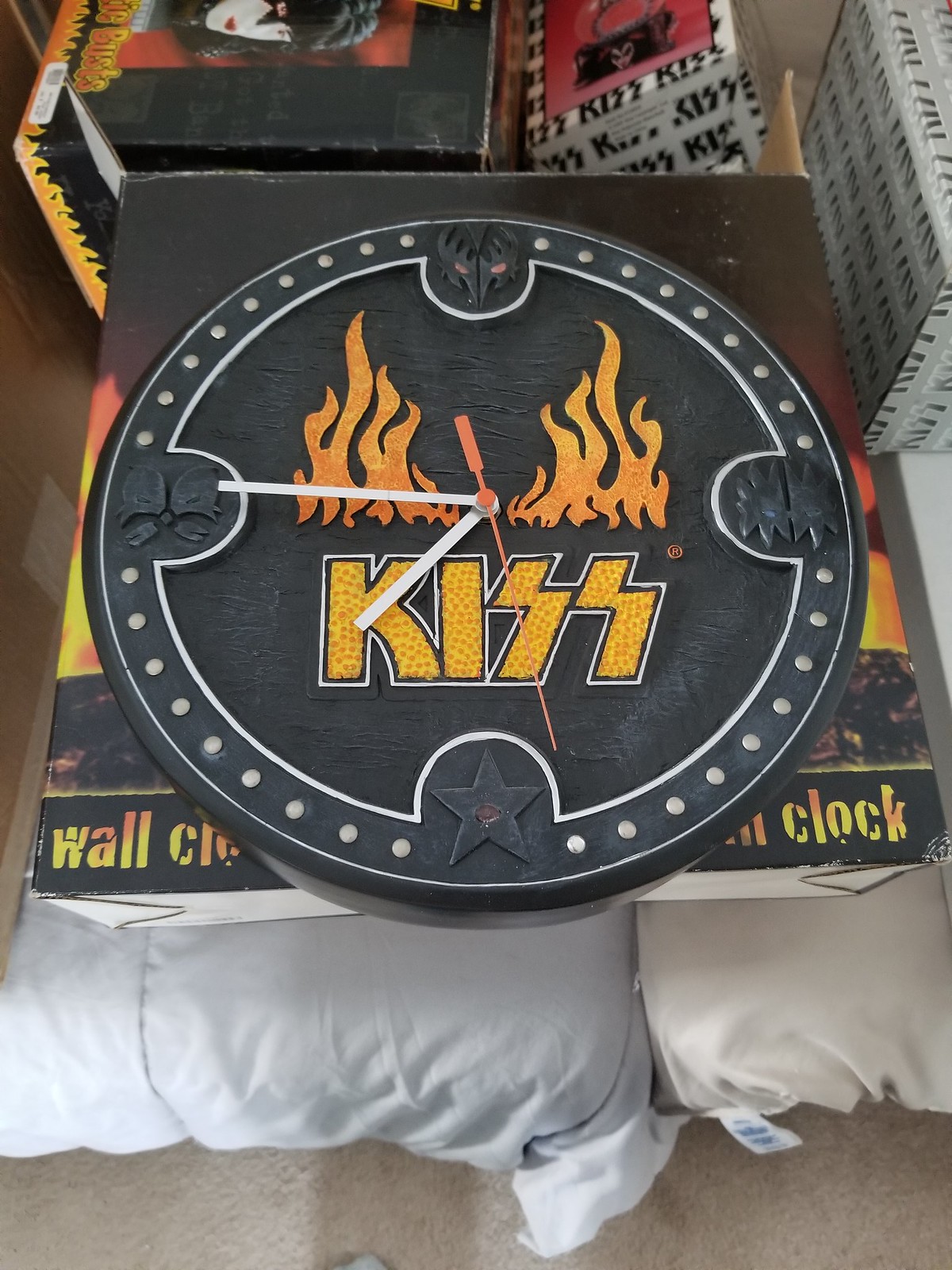The image showcases a striking KISS-themed wall clock, prominently featuring the iconic band's memorabilia. The clock itself is adorned with the KISS logo in bold gold lettering, set against a dramatic background of flames that frame the middle of the clock. This timepiece is distinctively designed with white hour and minute hands, a red second hand, and lacks numerical indicators. Instead, it features four unique graphics at the positions where the numbers 12, 3, 6, and 9 would typically appear: a wolf, a star, and two other black images. Encased within a box, the clock is accompanied by various other KISS memorabilia items. Below the clock, the text "wall clock in a box" is visible, suggesting its packaging. The box also contains additional KISS collectibles, including a small white box branded with the KISS logo and a graphic, and another worn black box featuring the face of a band member in their distinctive makeup. The entirety of this collection rests atop what appears to be pillows, adding a layered presentation to the ensemble.